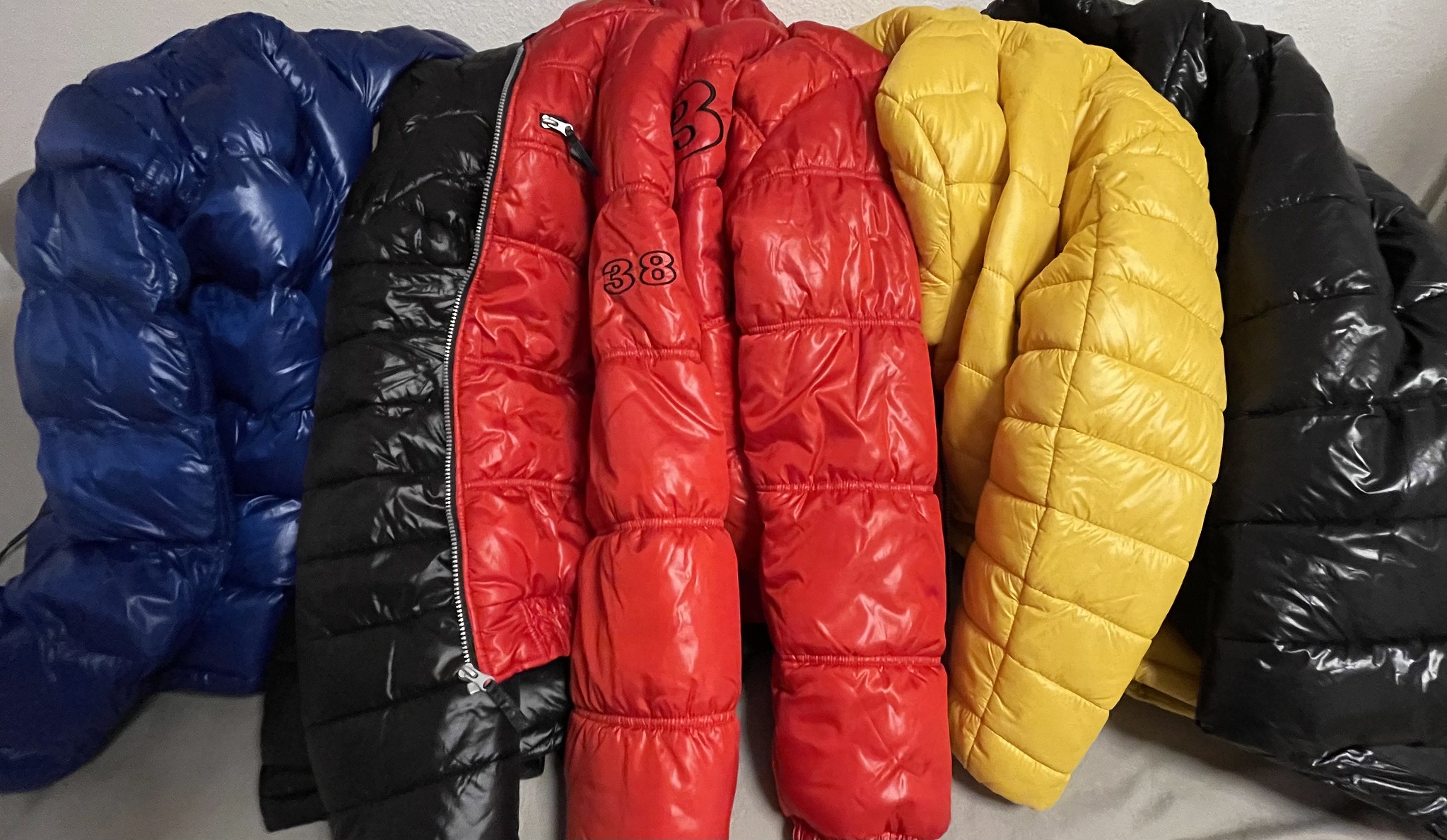The image displays an assortment of five puffy jackets arranged horizontally on a soft, beige-white cloth. Starting from the left, the first jacket is a dark blue, very puffy in material. Next to it is a distinctive jacket featuring a dual-color scheme of black on one side and red on the other, separated by a zipper. In the middle is a reddish-orange jacket labeled with the number "38," with part of an "8" visible on what would be the back, adding some uniqueness to the mix. The fourth jacket stands out with its bright yellow color, matching the puffy texture of the first jacket. Finally, the jacket on the far right is a solid dark black. All the jackets exhibit a shiny, pleather material, contributing to their plasticky appearance and emphasizing their puffed-up design, characterized by horizontal seams.